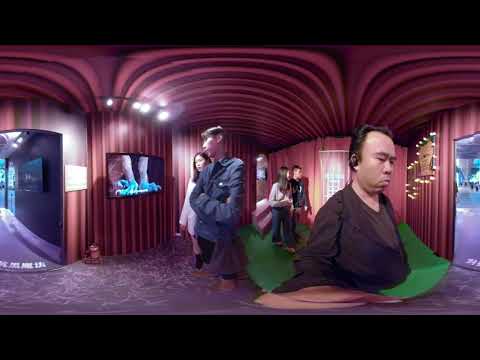The image is a distorted 360-degree photograph capturing a room with a strong fisheye effect. The setting appears to be a luxurious venue that might be a museum, theater, or a gallery, given its rich and elegant design. The walls and ceiling are covered in a magenta, wavy fabric-like texture that adds to the surreal and slightly disorienting atmosphere, reminiscent of a David Lynch film.

In the foreground, a man in his 30s, with slicked-back black hair and a black button-up shirt, is prominently holding a phone or camera. He wears headphones and looks deeply engaged, possibly listening to an audio tour. His figure appears unnaturally inserted into the room, only showing his upper half, adding to the surreal feeling.

Around him, there are two couples that seem unrelated. One couple, to the left, appears to be intently watching a screen, which displays a pair of green, bird-like feet with claws. The other couple is seen walking along the room, exploring the walls adorned with framed artwork and string lights. The space includes a staircase, contributing to the multi-dimensional feel of the area. Various entrances and exits suggest this might be a lobby or transitional space. The overall ambiance, with its luxurious and vibrant decor, feels both rich and otherworldly.